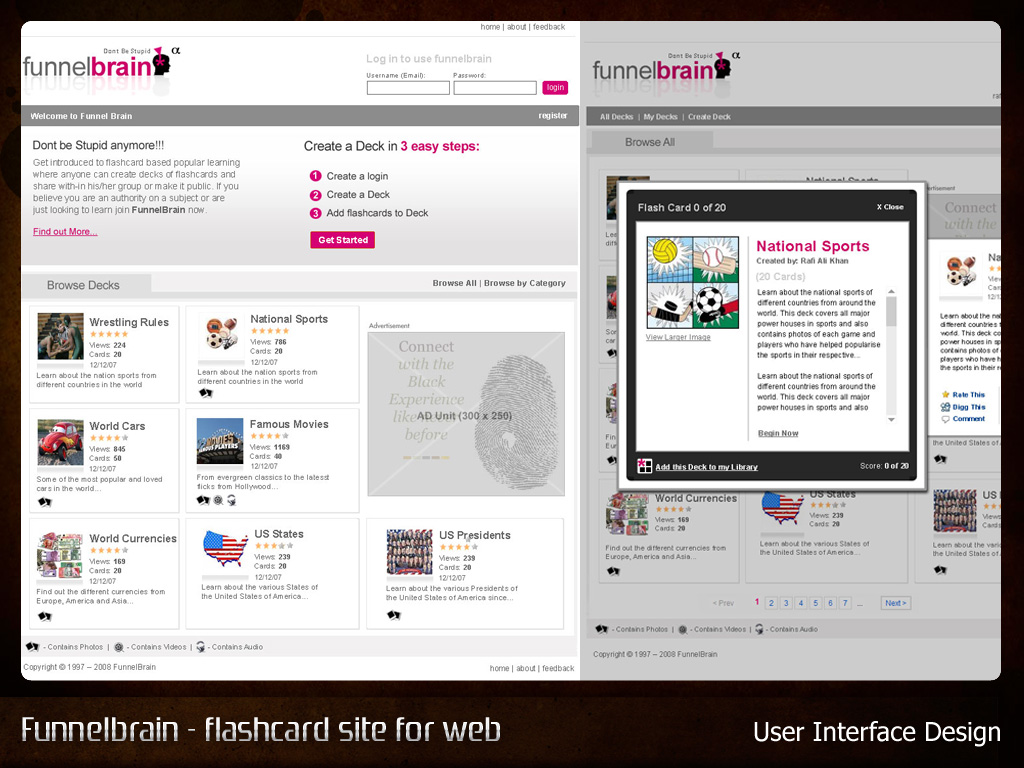The image showcases a user interface design for a web-based flashcard site named Funnel Brain, displayed prominently on the top left along with the slogan "Don't be stupid." The user interface is colorful and features a main banner encouraging users to "Create a deck in three easy steps: Create a login, create a deck, and add flashcards to the deck." The screen is divided into sections, one with a white background and another with a shadow gray background. 

The left section includes a logo depicting a side view of a human head with a pink star on top and a triangle emanating from it. Below the logo, there is a login area for users to enter their credentials. The site also presents various flashcard decks available for browsing, such as "Wrestling Rules," which contains 20 cards, "World Cars" with 50 cards, "World Currencies," "US States," "Famous Movies," "National Sports," and "US Presidents." 

The right section displays an example flashcard: "Flashcard 0 of 20" for the "National Sports" deck created by Rafi Ali Khan. It features a description of the flashcard deck and four images of different sports balls: a volleyball, a hockey puck, a baseball, and a soccer ball. Some user rankings, depicted as stars, and a small map of the US with a ship illustration can also be seen, adding to the educational and interactive nature of the page.